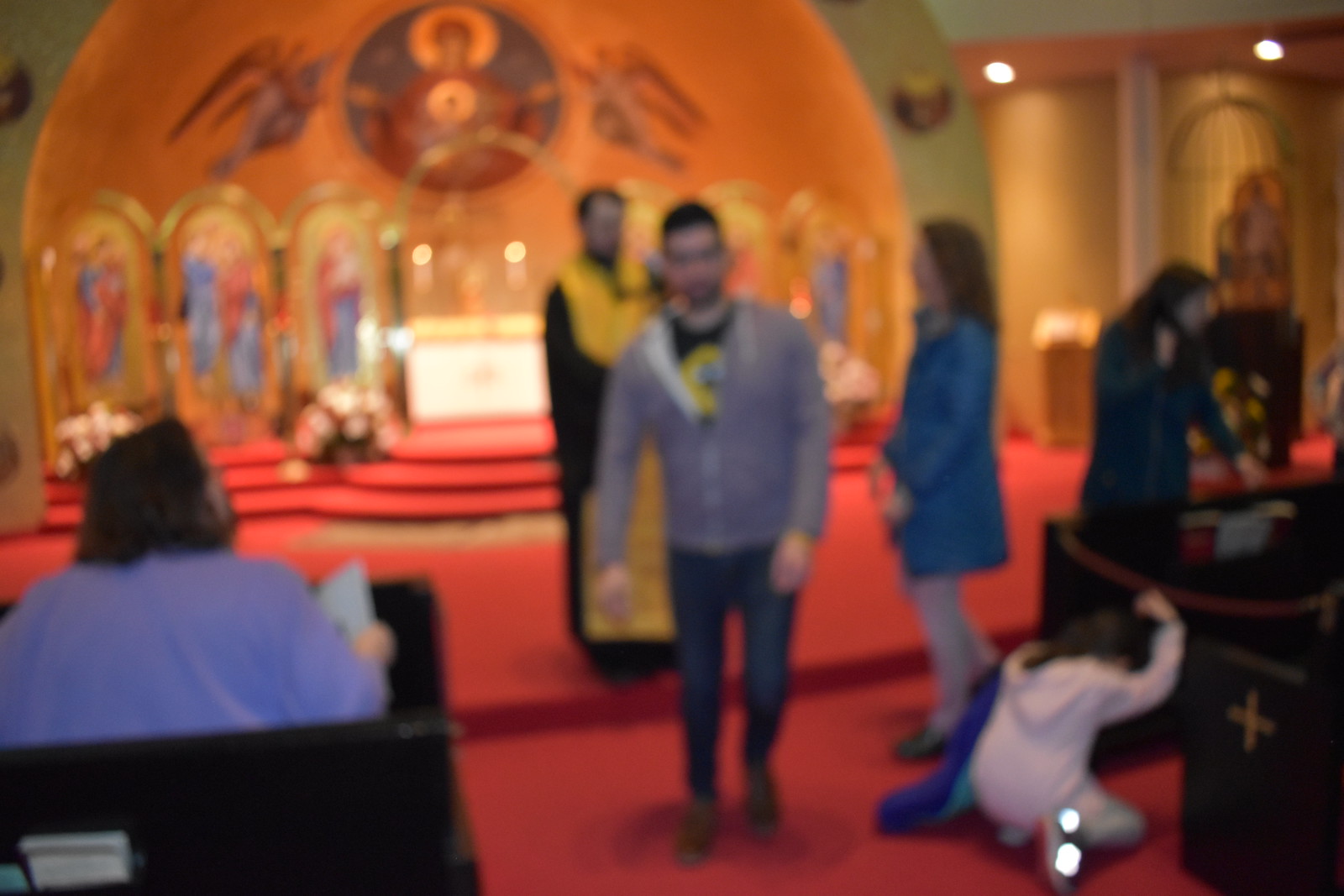A vibrant and bustling interior scene captures people moving about in a space that is somewhat out of focus and blurry. The atmosphere is brightly colored but lacks sharp delineation. On the left side of the image, a man with long hair, dressed in a strikingly bright blue shirt, sits in a high-backed black chair. In the center, a raised stage draped in layers of red catches the eye, initially appearing to host performers. However, upon closer inspection, the ceiling above displays religious icons, creating a juxtaposition that confuses the setting. The brightly lit environment feels atypical for a church, yet the religious iconography suggests otherwise, adding to the enigmatic nature of the scene.